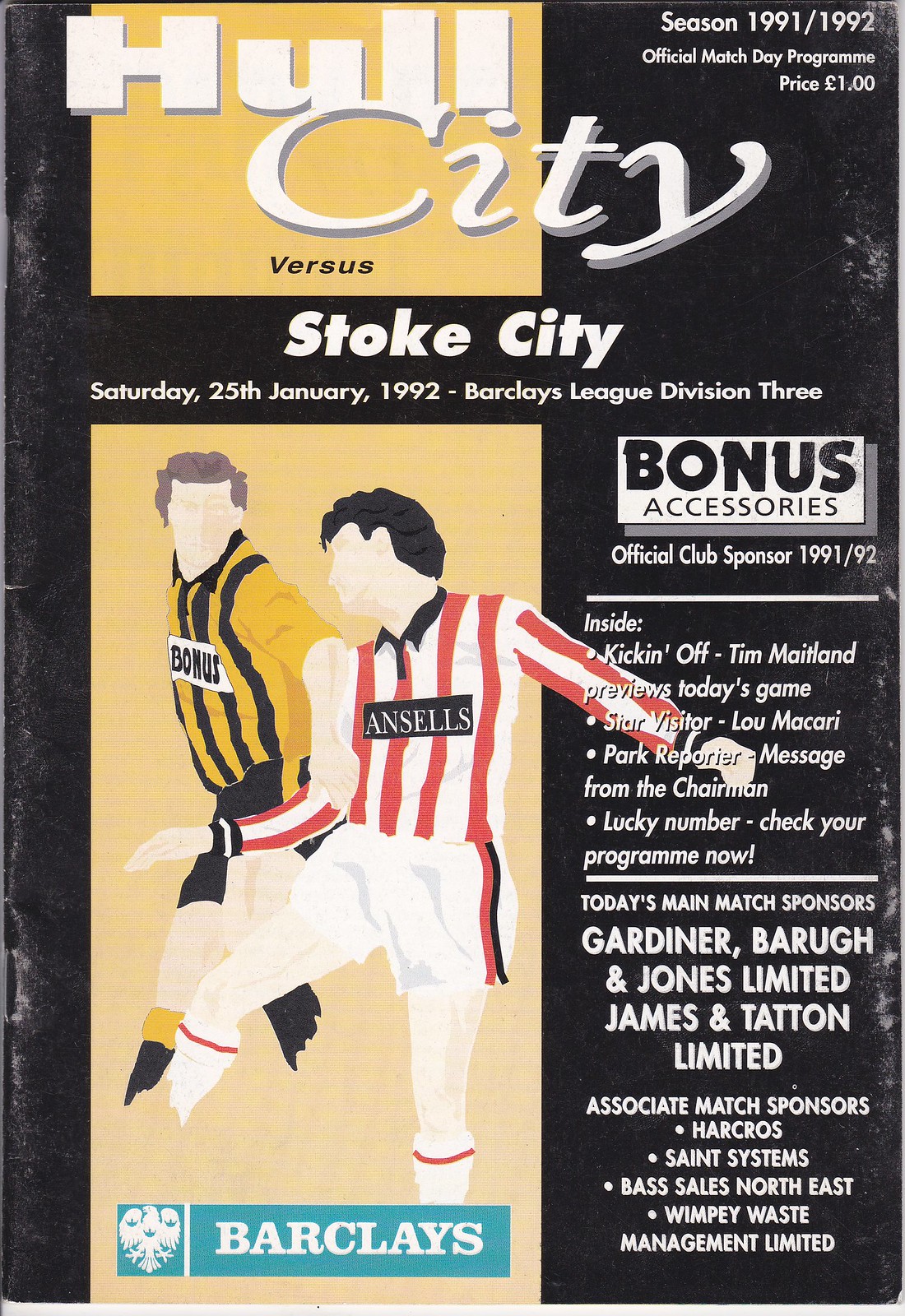The image depicts a match day program for a soccer game in England, specifically between Hull City and Stoke City, from the 1991-1992 Barclays League Division III season. The program, priced at £1, is for the match held on Saturday, January 25, 1992. The background is predominantly black with most of the text in white font. At the top of the program, large white lettering announces "Hull City vs. Stoke City." In the upper right corner, it specifies "Season 1991-1992 Official Match Day Program."

Near the center, there is a cartoon-like illustration of two soccer players on a yellowish background. The player on the left, with light brown hair, is dressed in a white and red kit with the word "Bonus" on the jersey, while the player on the right, with black hair, wears a red and white striped jersey that says "Ansel's" and white pants with red and black trim. The image cuts off at their legs, omitting their feet. 

At the very bottom of the program, there is a blue and white Barclays logo, featuring a bird emblem. To the right of the player images, additional text details the main match sponsors and highlights from the program, including: 
- "Bonus Accessories Official Club Sponsor 1991-92"
- "Kicking Off: Tim Maitland previews today's game."
- "Star Visitor: Lou Macari"
- "Park Reporter: Message from the Chairman"
- "Lucky Number: Check your program now."

Additionally, it lists today's main match sponsors: "Gardner Barrow & Jones Ltd., James & Tatton Ltd.," and associate match sponsors: "Harcrows, St. Systems, Bass Sales Northeast, Wimpy Waste Management Ltd."